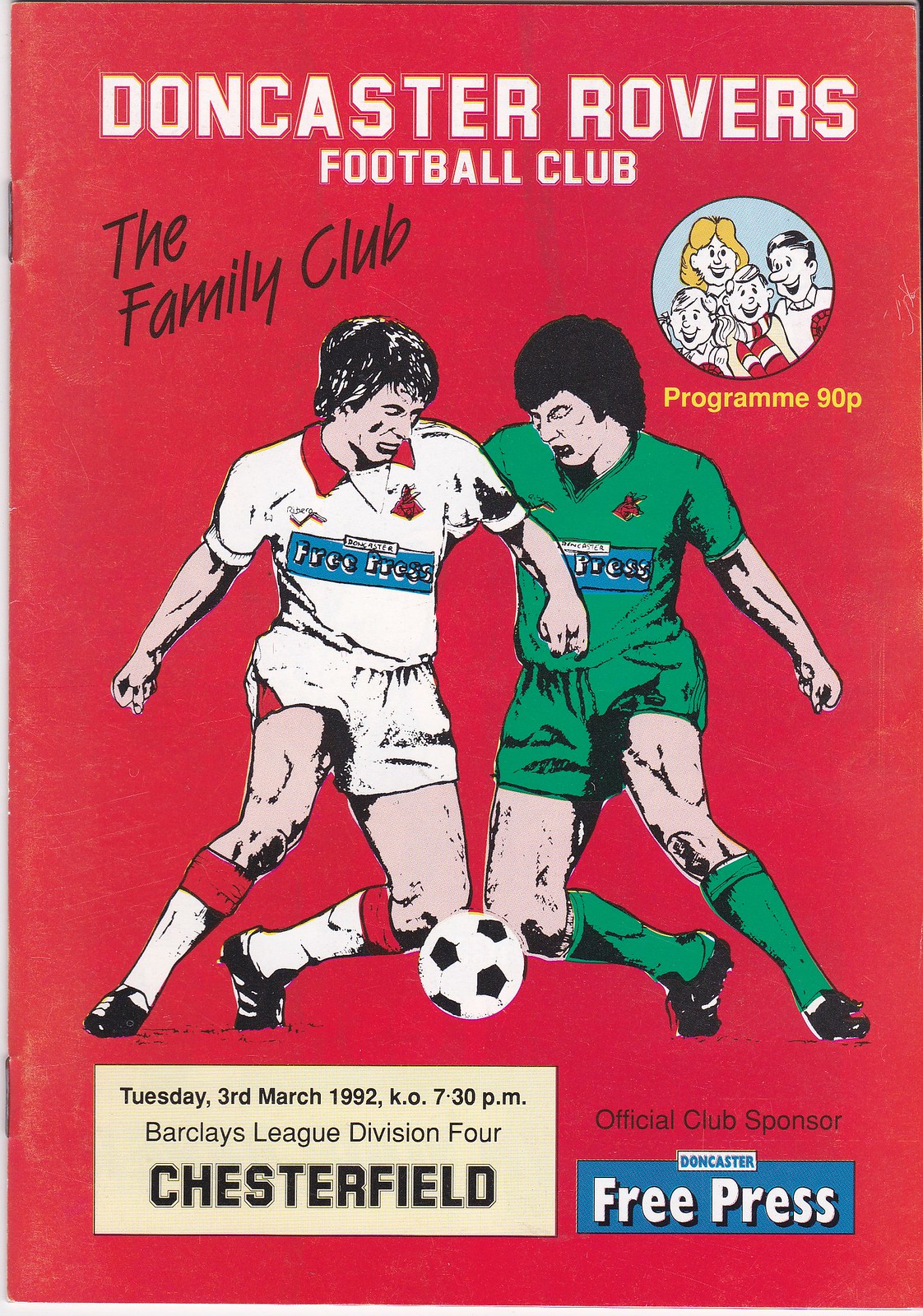This image is an old, grainy poster, likely taken from a magazine or comic book, advertising the Doncaster Rovers Football Club. The poster features a faded red background. At the top, bold white text with a light red outline reads "Doncaster Rovers," and beneath it, in smaller white print, it says "Football Club." Below this, slanted from the lower left to the upper right in black, stylized text, it says "The Family Club." To the right is a circle with a blue background containing a cartoon drawing of a family of four: a dad with a long nose and black hair, a blonde mom in the background, and two children in front. Below the circle, yellow text reads “Programme 90P.”

The main image depicts two soccer players vying for a ball at their feet. The player on the left is dressed in a white short-sleeve jersey with a red collar, white shorts, white socks with red stripes, and black shoes. His shirt features a blue rectangle with the white text "Free Press." The player on the right wears a green jersey, presumably with a similar blue rectangle on his shirt that is partially obscured, wearing black shoes. 

In the bottom left corner, a large horizontal light brown rectangle contains the event details in black text: "Tuesday, 3rd March 1992, K.O. 7.30 p.m., Barclays League Division IV, Chesterfield." The bottom right corner features the phrase "Official Club Sponsor" in black print. Beneath it, a blue rectangle with a small white rectangle attached to its center contains blue text "Doncaster" and white text "Free Press," reflecting the sponsor's logo.